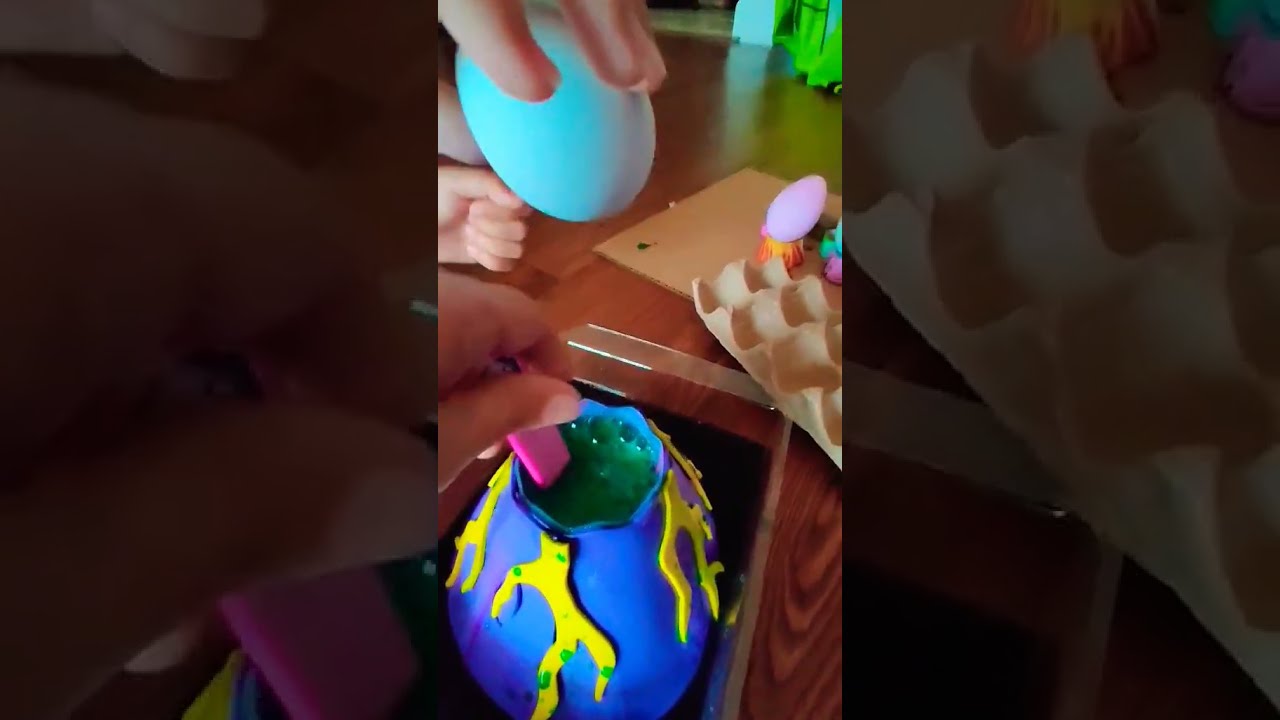The image shows an array of hands engaging in a craft activity centered around intricately decorated eggs. Dominating the foreground is a deep bluish-purple egg, potentially made from clay or plastic, adorned with raised yellow markings resembling seaweed. A foaming green substance inside the egg is being stirred by a pink spoon. Nearby, another hand holds a turquoise egg above what looks like a science project resembling a miniature blue and yellow volcano filled with green liquid. In the backdrop, an egg carton containing more of these uniquely shaped and decorated eggs is visible, with tiny hands reaching into it. The setting appears to be a kitchen table amidst a blurred, colorful room, adding an artistic and somewhat mysterious atmosphere to the image.